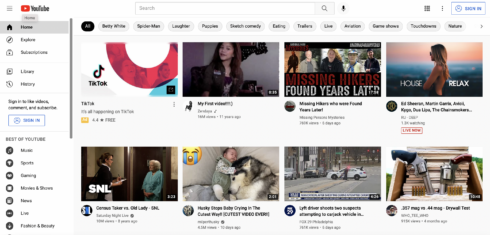The image is a screen capture of a YouTube page, viewed on a desktop computer. In the upper left corner, the iconic YouTube logo is prominently displayed. Directly below the logo, an array of YouTube links and menu options are aligned vertically. The "Home" icon is distinctly highlighted with a grey bar, indicating its active status.

On the right side of the menu, eight video thumbnails are organized in a tidy grid of two rows, each containing four video links. 

In the top row, the very first video thumbnail on the left features content related to TikTok. This thumbnail is visually striking with a red semicircle design paired with a blue design element.

Directly below this, in the second row, the first video thumbnail showcases a scene from "Saturday Night Live" (SNL). The foreground of the image captures a woman wearing a black outfit, with "SNL" boldly emblazoned in white letters across her attire.